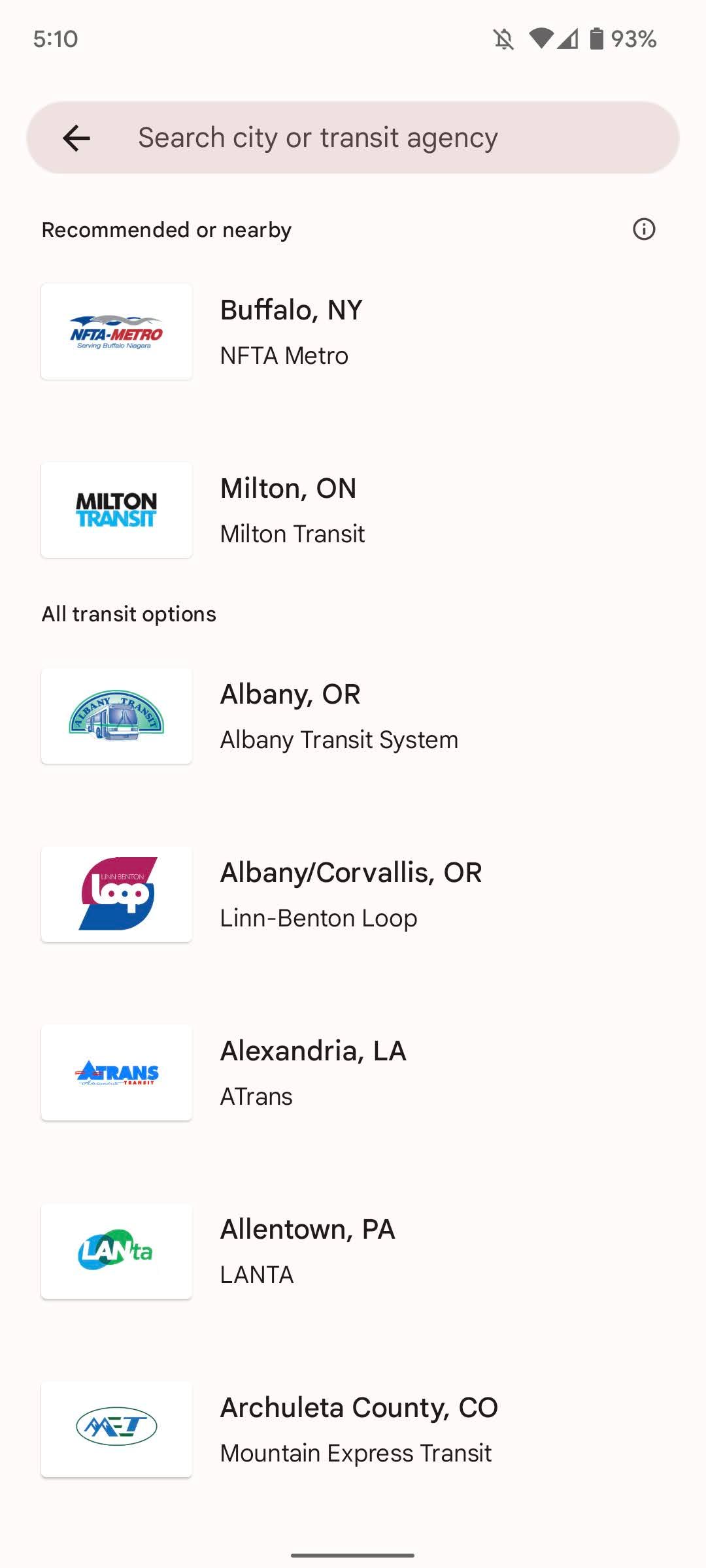This image is a screen capture of a smartphone application listing various city or transit agencies. In the upper right-hand corner, the battery icon displays 93% power remaining, and the cell service indicator shows almost full bars. The Wi-Fi is fully connected, and there is no active alarm, as indicated by the alarm icon being off. In the upper left-hand corner, the time is displayed as 5:10.

The background color of the app is a soft whitish-peach hue. Directly below the top bar is a search area featuring a back arrow on the left and the text "Search city or transit agency." Below the search area, the app displays the section "Recommended or Nearby" with an eye icon enclosed in a circle to the right.

Under this section, several transit options are listed:
1. **Buffalo, New York** - NFTA Metro, accompanied by the NFTA Metro logo.
2. **Milton, Ontario** - Milton Transit, with the Milton Transit logo.
3. **Albany, Oregon** - Albany Transit System, with the Albany Transit logo.
4. **Albany/Corvallis, Oregon** - Linn-Benton Loop, alongside the Loop logo.
5. **Alexandria, LA** - ATrans, with the ATrans logo.
6. **Allentown, PA** - Lanta, including the Lanta logo.
7. **Archuleta County, Colorado** - Mountain Express Transit (MET), accompanied by the MET logo.

At the bottom of the list is a section labeled "All transit options," indicating additional choices available within the app.